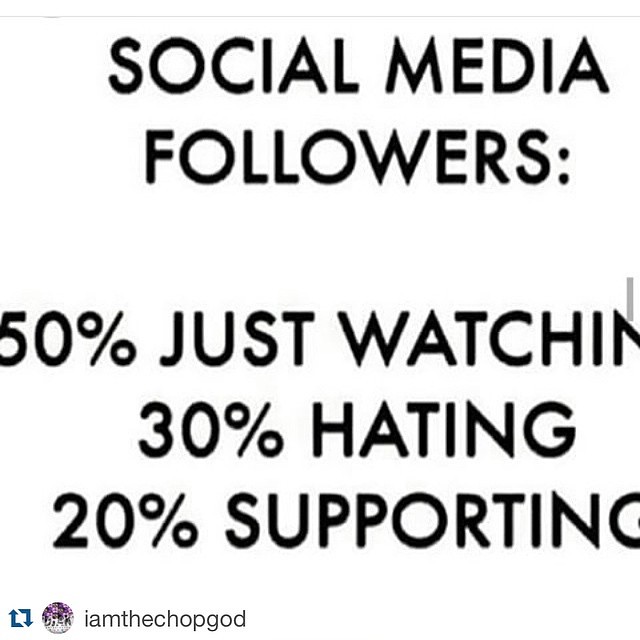The image is a widely circulated, low-resolution Instagram post featuring a black text meme on a white background. The centered, all-caps black font reads: "SOCIAL MEDIA FOLLOWERS: 50% JUST WATCHING, 30% HATING, 20% SUPPORTING." In the bottom left corner, there is a round logo with purple, white, and blue elements beside a square icon formed by two blue arrows, indicating the use of a repost app. Beneath this, in lower case and black font, is the username "i am the chop god." This composition implies the content has been repeatedly saved and shared across social media platforms.